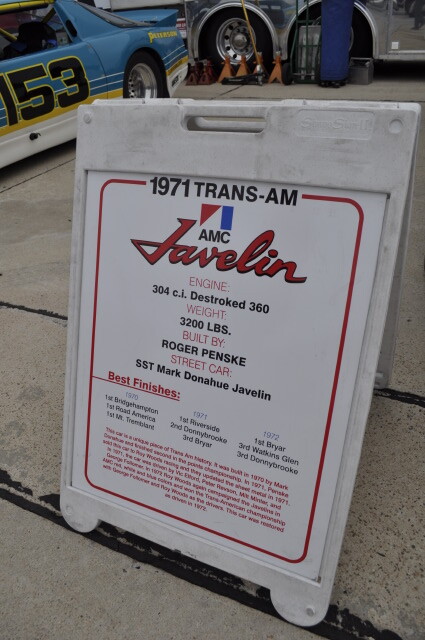The image features a plastic banner on the ground, displaying detailed information about a race car. At the top, in bold black letters, it reads "1971 Trans Am." Beneath this, it highlights the car's make and model as an "AMC Javelin," with further details including "Engine: 304 CI D Stroke 360" and "Weight: 3200 Pounds." The banner credits "Built by Roger Penske" and identifies the car as a "Street Car SST Mark Donahue Javelin." There is also a larger paragraph in very small print that is unreadable. The banner’s design includes various colored shapes: a red triangle, a white triangle, and a blue rectangle. In the background, a powder blue race car with yellow stripes, bearing the number 153 and the name "Peterson" in yellow, can be seen. The car, which has older styling indicative of its 1971 vintage, sits on a gray sidewalk with black lines. Adjacent items, such as automobile parts and a small silver pail, further accentuate the race-ready ambiance of the scene.